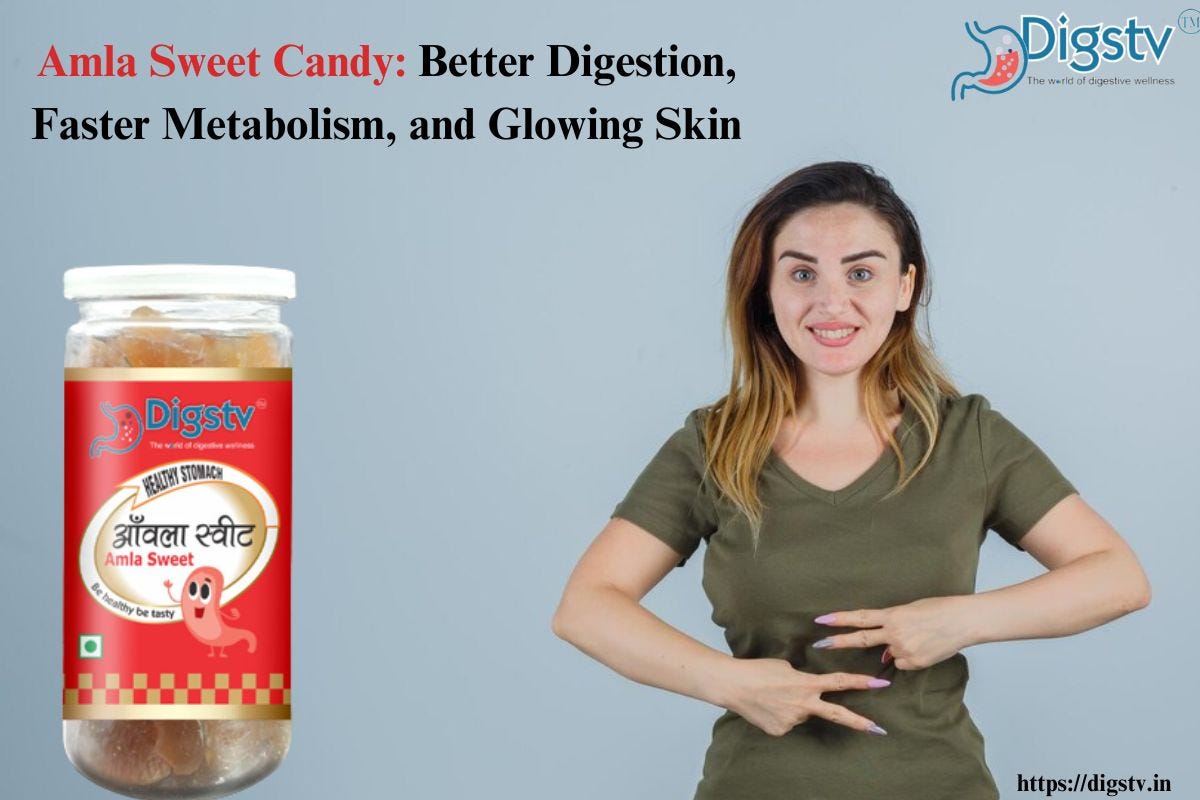This striking advertisement features a young woman with dark hair transitioning to blonde tips, smiling and flashing peace signs over her stomach. She wears an olive green short-sleeved shirt against a soft blue background. At the top left, bold red text spells "Amla Sweet Candy," followed by black text detailing the benefits: "Better Digestion, Faster Metabolism, and Glowing Skin." Adjacent to this, a small illustration of a stomach filled with pink acid and bubbles is labeled "DIGSTV, The World of Digestive Wellness." At the bottom left, a transparent glass jar with a white lid and a vibrant red label showcases gummies. The label reads "DIGSTV," "Healthy Stomach," and "Be Healthy, Be Tasty," accompanied by a cheerful cartoon stomach character. The edges of the label feature a red and gold checkered pattern, and the bottom right corner of the ad discreetly presents the website link "HTTPS://DIGSTV.IN."